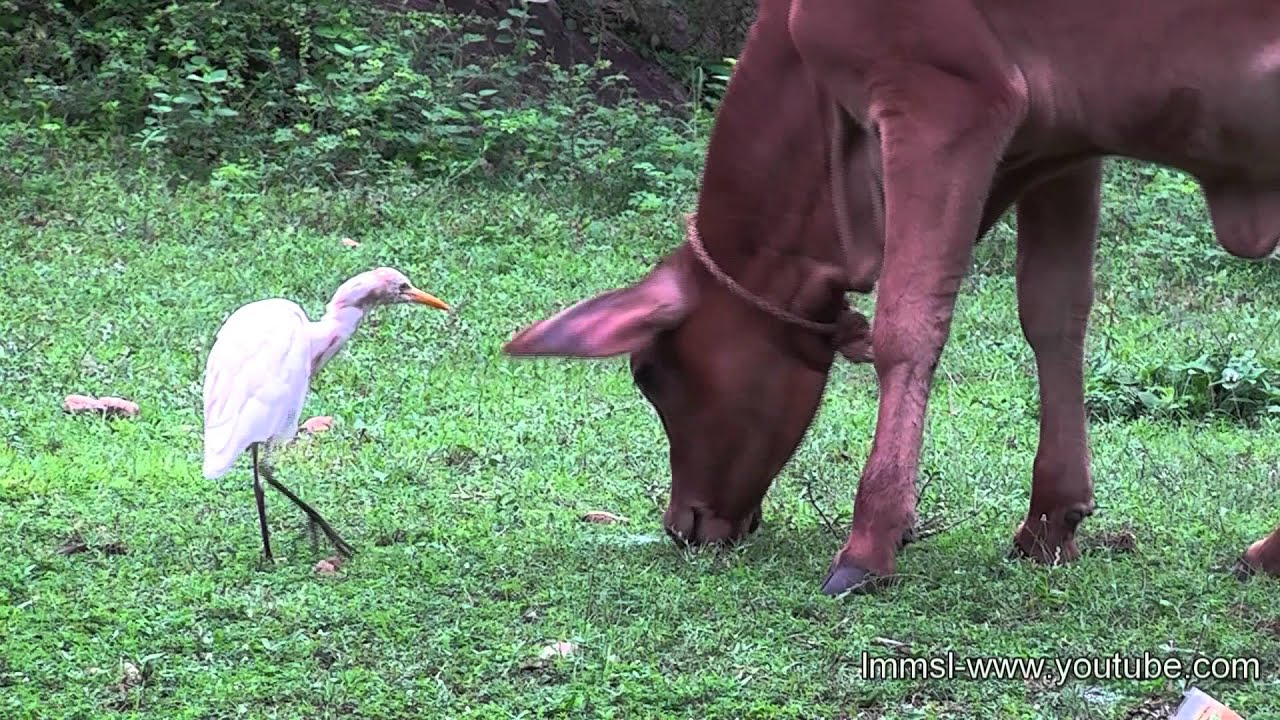This detailed photograph features a brown cow, possibly a female as part of its udder is visible on the right edge of the image, standing or grazing in a lush area with abundant green grass. The cow has a brown necklace or rope around its neck with white lettering that reads "LMMSL-W-WWW.YOUTUBE.COM." Nearby, towards the left of the cow, there is a white cattle egret. The egret is slender, with long, skinny black legs and an elongated yellow beak. It appears to be gazing attentively at the cow, possibly at its ear. The setting includes taller bushes or trees in the background, enhancing the scene with natural elements.